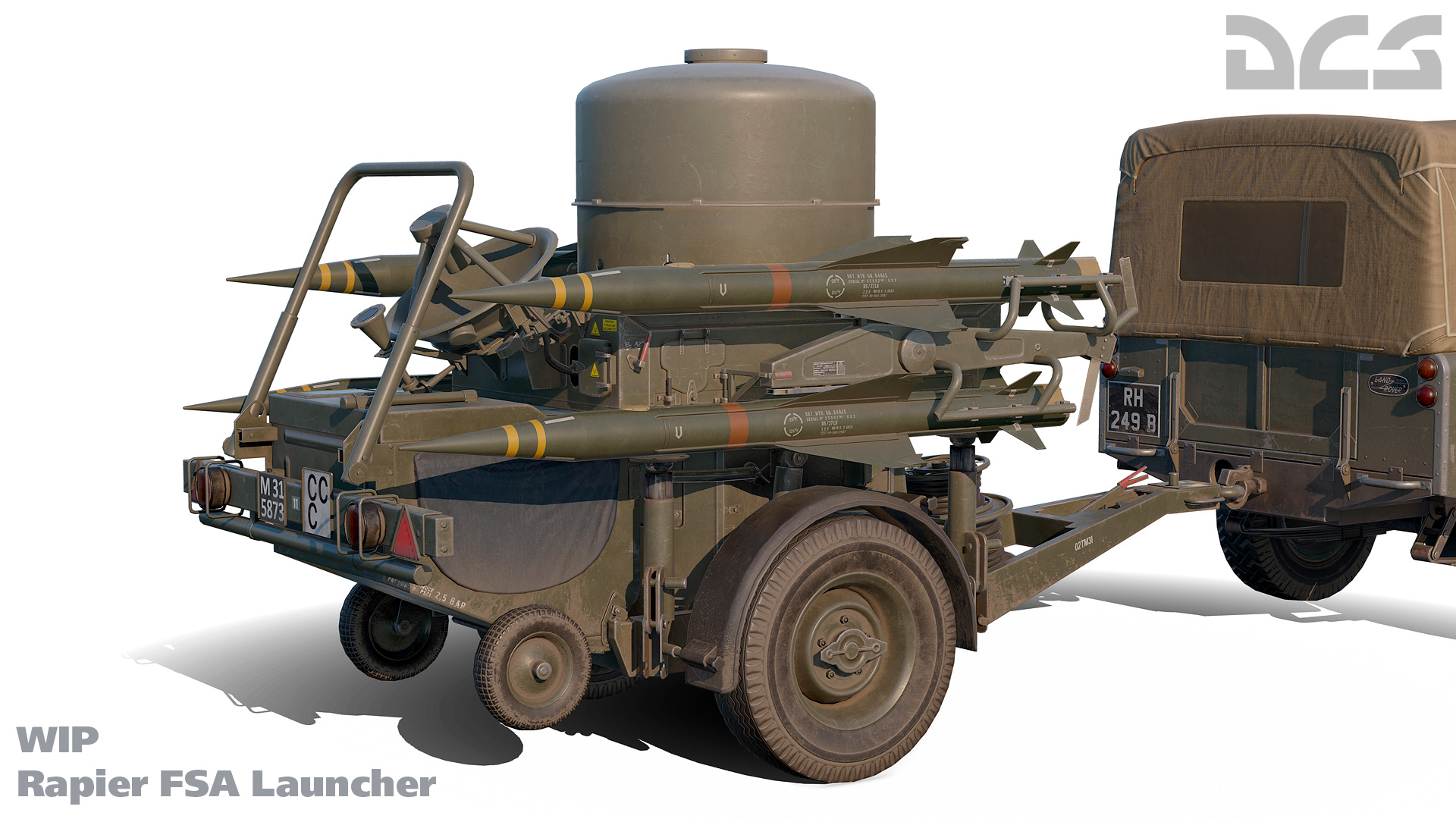The image showcases a 3D rendering of a green military jeep-like truck with a canopy cloth roof, pulling a trailer laden with weaponry. The truck, identified by a black license plate with white lettering "RH249B," is viewed from the back with much of its outer frame visible. Connected via a trailer hitch, the trailer rests on two large black wheels, with two smaller wheels suspended in the air. Central on the trailer is a round barrel-like cylinder, flanked by two sets of missiles on either side—four in total—each equipped with fins and pointed tips. The entire scene is set against a backdrop of assumed military context, possibly educational or indicative of wartime activity, indicated by the positioning of the vehicle and its armament. In the bottom left, the text "WIP Rapier FSA Launcher" is displayed, suggesting an in-progress repair or construction of the launcher system. The color palette includes shades of green, black, white, gray, tan, brown, yellow, and red.